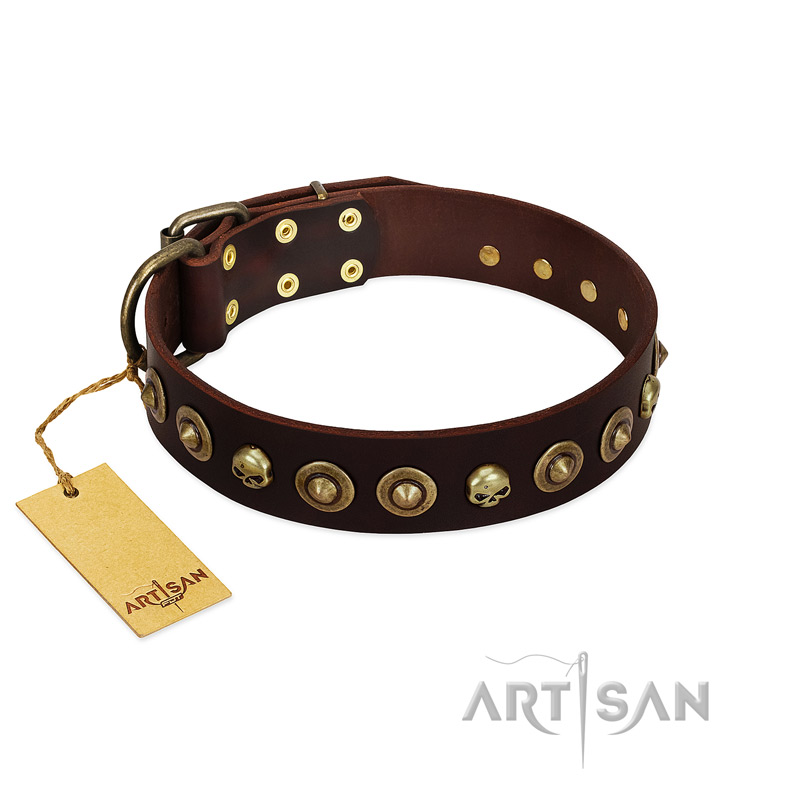The image features a brown leather accessory, which could be either a collar or a belt, set against a plain white background. The accessory is adorned with brass skull studs and pointy-tipped studs arranged in a pattern around it. It is partially wrapped, displaying both the exterior and interior of the leather piece. There is a cardboard tag attached to the accessory with a string, positioned towards the bottom of the image. The tag and the bottom right corner of the image both feature the brand name "ArtSan," with a design where a needle and thread replace the letter "I." The image focuses on the intricate detailing of the hardware and the artisanal craftsmanship of the accessory.